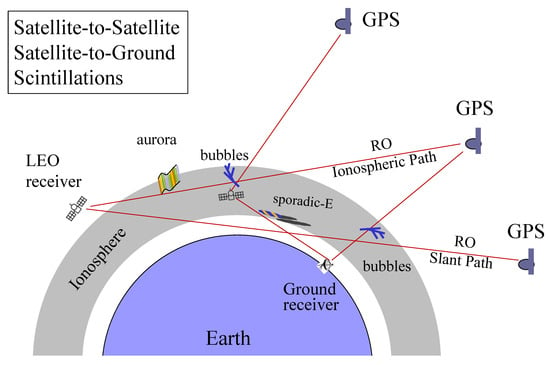This detailed diagram illustrates satellites beaming information to Earth against three main layers. At the bottom is a semi-circular, blue section labeled "Earth," outlined in black. Above Earth is an unlabeled white layer, and above that is a gray, semi-circular section titled "Ionosphere." The graphic shows various satellites, including GPS and LEO receivers. 

In the top left corner, there is a black rectangle with white text reading "Satellite to Satellite, Satellite to Ground, Scintillations." Red lines traverse the diagram, connecting satellites to different points, such as "Ground Receiver," "Aurora," "Bubbles," "RO," "Ionoshperic Path," and "Sporadic E." One notable path leads from the "LEO Receiver" across to "RO Slant Path" and "GPS." Overall, the diagram is a complex visualization of how satellite signals move between the Earth and different atmospheric layers, highlighting key components and interaction points in the transmission process.